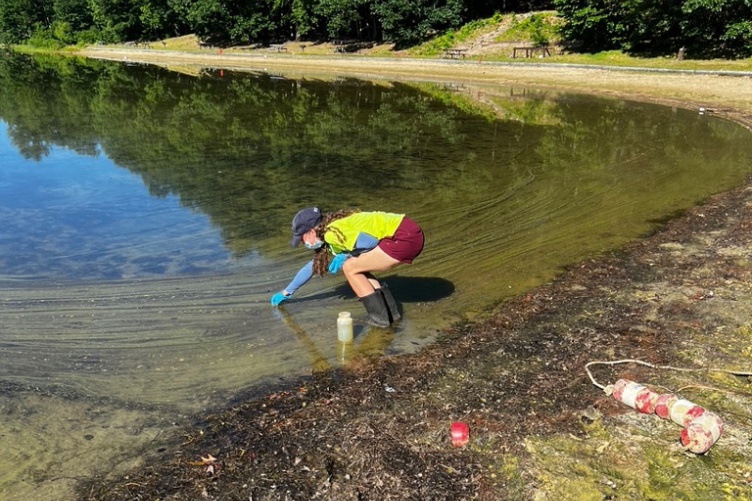In a color photograph of a serene lake or pond, a woman, appearing to be an environmentalist, is meticulously collecting water samples. Standing at the muddy shore which transitions into dark, algae-infested waters, she is hunched over and reaching her gloved hand into the lake. She wears black boots, maroon shorts, a neon yellow t-shirt, a blue baseball cap, and protective blue gloves. Adjacent to her on the muddy ground lies a small white canister, presumably for storing the collected samples. Behind her, patches of brown dirt and vegetable matter scatter the shore. Further back a red and white buoy and some unidentified red plastic pieces linked by a string are visible. In the distance, a walking path meanders around the lake, flanked by benches. The surrounding foliage and blue sky are beautifully reflected in the murky water, highlighting the environmental essence of the scene. Some descriptions mention the woman wearing a face mask, underlining the seriousness and perhaps the safety measures involved in her task.